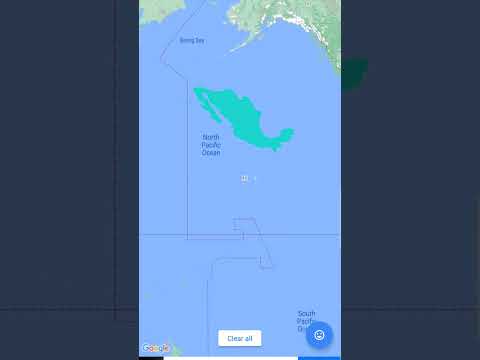A screenshot from Google Maps features a detailed view of a small island situated in the North Pacific Ocean. The island is marked in green and positioned below a larger landmass that extends into the ocean with a prominent peninsula or jetty. The ocean is divided into sections by lines, and the South Pacific Ocean is labeled in the bottom-right corner. Additional map interface elements include an option to clear all, a blue circle with a smiley face in the bottom-right corner, and the Google watermark in the bottom-left corner. The map display occupies the central portion of the screen in a narrow rectangular format, with black sections on both sides. The landmass in the image is depicted in shades of green and white.